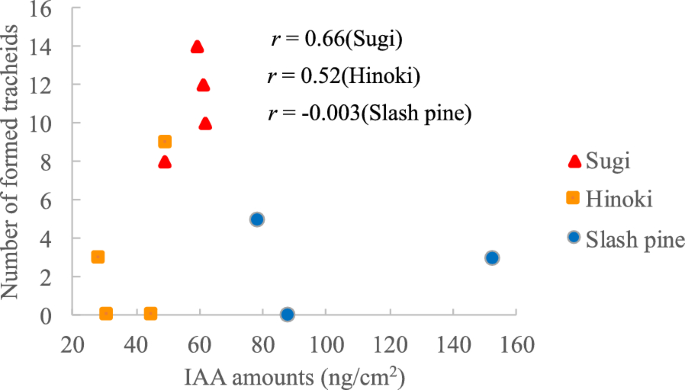The image depicts a detailed, professionally-made graph with a white background. The graph has a vertical Y-axis labeled "Number of Formed Tracheids," ranging from 0 to 16 in increments of 2. The horizontal X-axis is labeled "IAA Amounts (NG/cm²)," ranging from 20 to 160 in increments of 20. 

Scattered throughout the graph, there are three distinct symbols: red triangles, yellow squares, and blue circles, representing "sugi," "hinoki," and "slash pine," respectively. In the upper right-hand corner, three italicized R-values are provided: R = 0.66 (sugi), R = 0.52 (hinoki), and R = -0.003 (slash pine). These points are plotted against the axes grid, visually correlating the number of formed tracheids with varying IAA amounts for the different tree types.